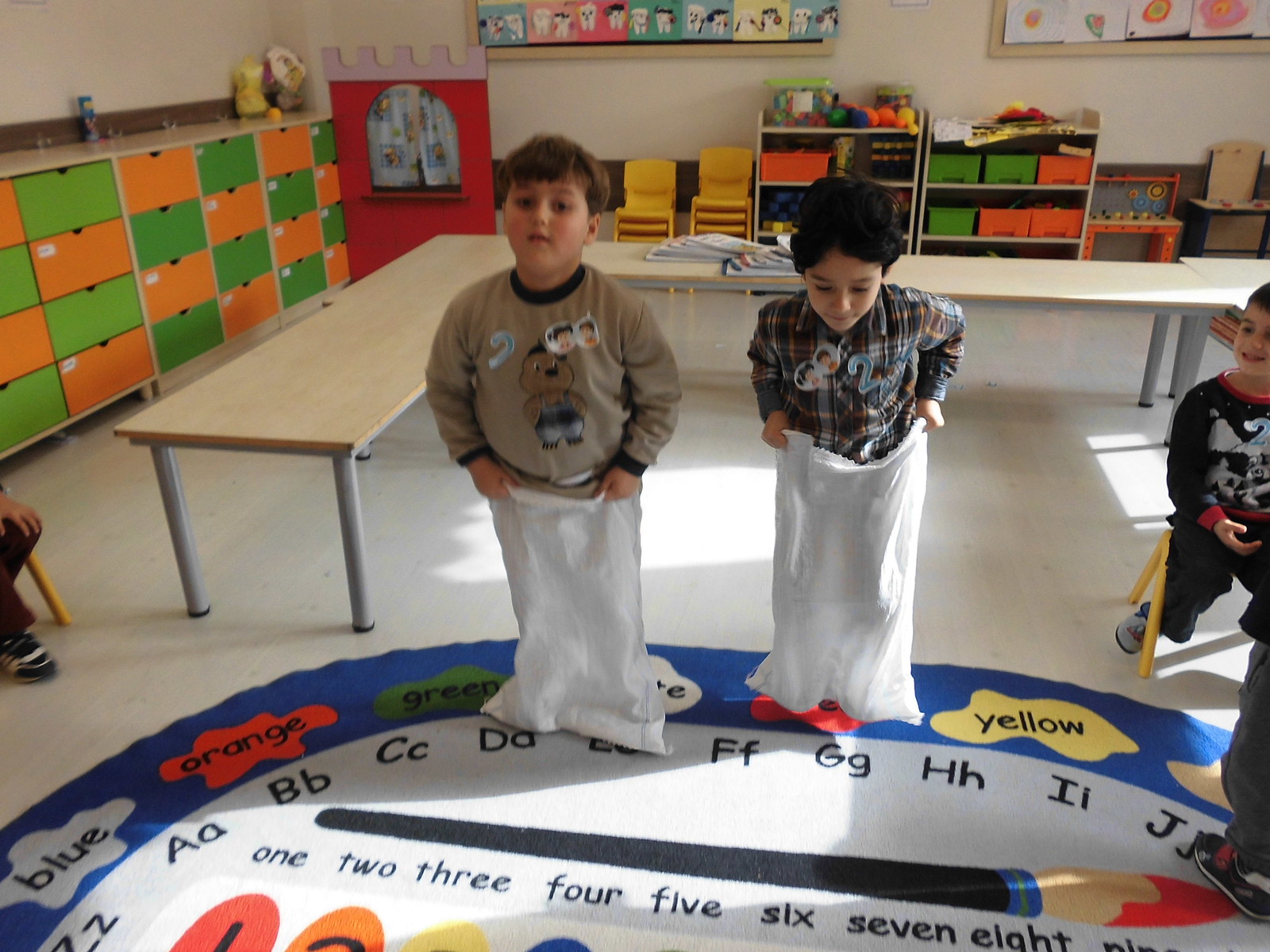In a brightly colored kindergarten or preschool classroom, four boys are captured in various activities. Two boys, partially visible in the frame, stand on a large circular rug adorned with the alphabet and vivid paint splotches in colors like blue, green, orange, red, white, and yellow. The rug also features the numbers 1 through 9 beneath a large paintbrush graphic. These two boys appear ready for a sack race, each holding up a white beanbag sack to their waists. One boy gazes directly at the camera while the other looks down. To the right, the legs of a fourth child sitting on a chair are visible, suggesting a lively, engaged environment. The classroom is filled with green and orange cubbies, yellow chairs, and colorful pictures on the wall, further enhancing the cheerful, educational setting.